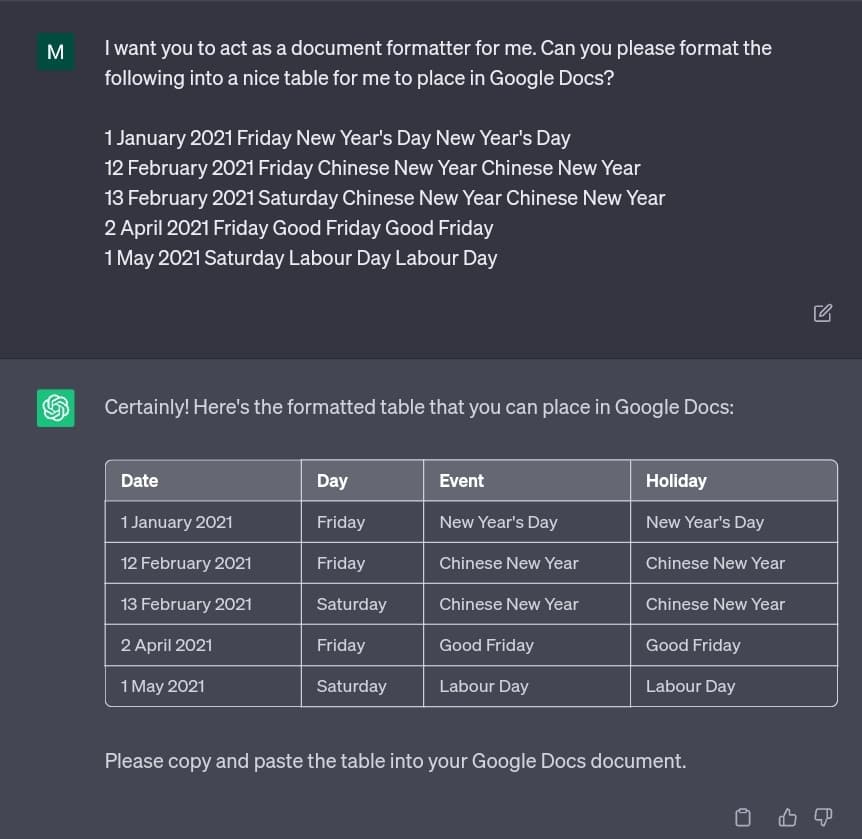This image is a screenshot showcasing a dialogue on ChatGPT, structured horizontally into two halves: a dark gray top half and a medium gray bottom half. The top half features a square icon with a green background and a white "M" located in the upper left corner. To the right of this icon, white text reads: "I want you to act as a document formatter for me. Can you please format the following into a nice table for me to place in Google Docs? 

1 January 2021, Friday, New Year's Day, New Year's Day.
12 February 2021, Friday, Chinese New Year, Chinese New Year.
13 February 2021, Saturday, Chinese New Year, Chinese New Year.
2 April 2021, Friday, Good Friday, Good Friday.
1 May 2021, Saturday, Labor Day, Labor Day."

In the bottom half, the ChatGPT icon is positioned in the upper left corner, followed by text that reads: "Certainly, here's the formatted table that you can place in Google Docs." Below this response is a neatly formatted table containing the provided information. At the very bottom, a final line of text instructs: "Please copy and paste the table into your Google Docs document."